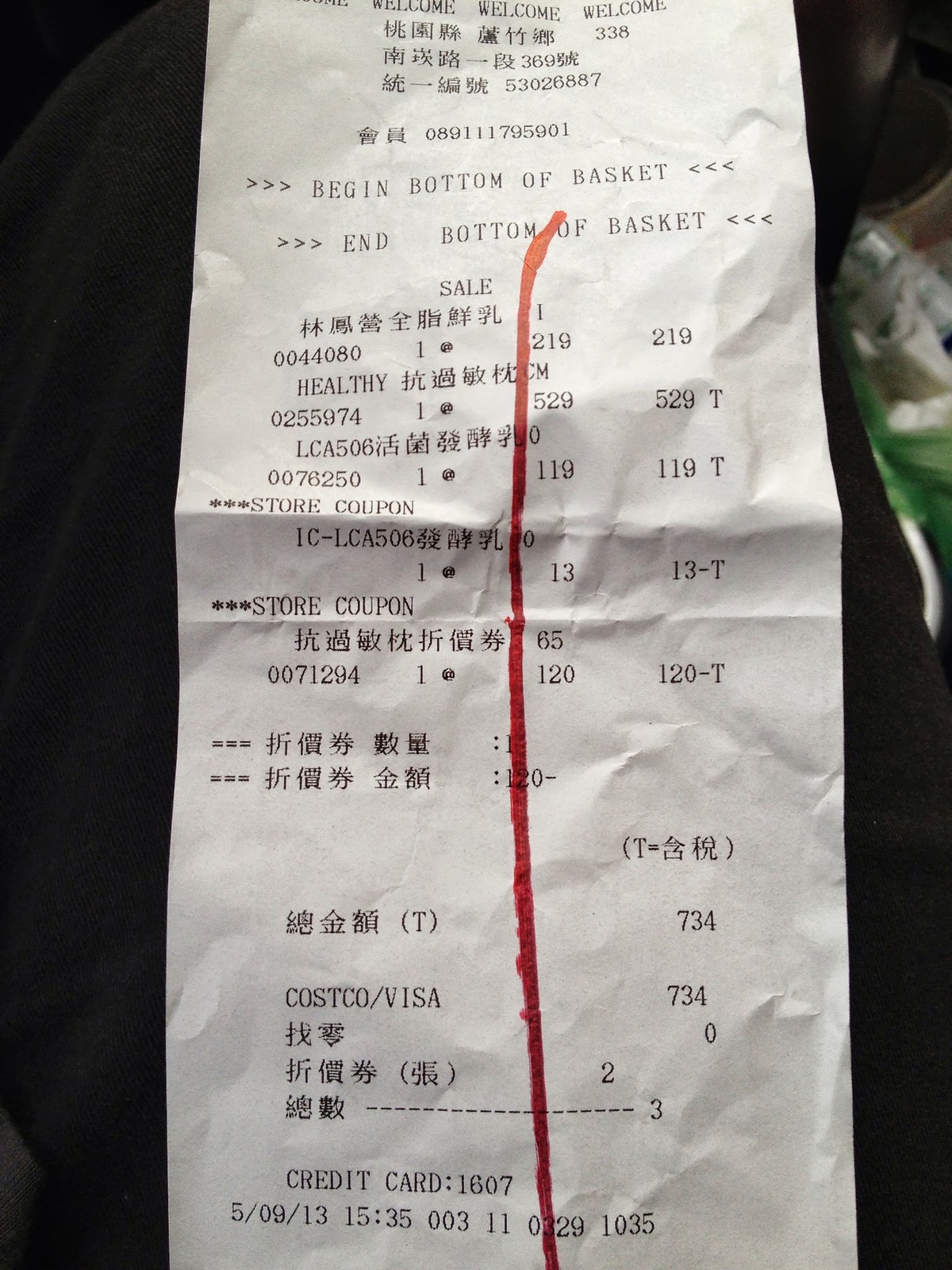This is a photograph of a white Costco receipt against a predominantly black background, with a touch of white and green appearing in the top right corner. The receipt appears to be in Japanese, though a few phrases in English are visible. At the top, the receipt warmly greets with "WELCOME, WELCOME, WELCOME." Notably, there are English phrases "BEGIN BOTTOM OF THE BASKET" and "END BOTTOM OF THE BASKET" printed along the list of items. A prominent red marker line runs vertically down the center of the receipt, adding a striking contrast to its white paper. At the very bottom, the text "CREDIT CARD... 1607-509-13" is discernible, indicating payment details.